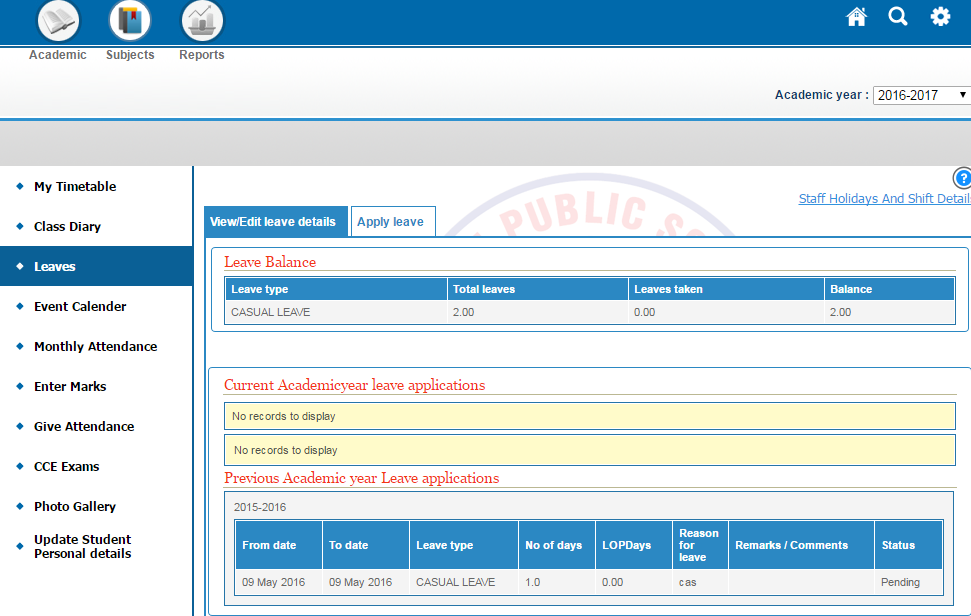The image depicts a school-themed interface with distinct sections and icons, providing an organized academic overview. At the top, there's a dark blue border spanning the width of the image. On the left side, several circular icons are aligned vertically: 

1. The first circle features an open book on a blue background.
2. To its right, a circle contains a blue square set against a white background.
3. Another circle depicts an arrow above three books on a light blue background.

Moving rightwards, the interface displays a series of white icons on a light background, aligned horizontally:
- A settings icon
- A search icon
- A home icon

Above, there's a light blue border, transitioning to a light gray border. Below these icons, the text "Academic and Subjects" and "Reports" appears in black. Just below, on the right side, there's a label "Academic Year" within a small white rectangle, indicating "2016 to 2017." Beneath this, a thin blue line runs horizontally across the section.

To the left side, nine small blue diamonds are arranged vertically. Adjacent to these diamonds, clickable black text elements are listed, with the third item labeled "Leaves" highlighted by a blue bar.

A detailed panel appears on the right, containing two tabs: a blue one labeled "View/Edit Leave Details" in white text, and a white tab labeled "Apply Leave" in blue. Below this, there's an underlined section titled "Staff Holidays and Shift Detail" in blue text, accompanied by a blue circle with a white question mark.

To the left, beneath the blue and white tabs, titled "Leave Balance," several blue tabs with white text contain subcategories. Further down, additional information in black text is organized, leading to the section titled "Current Academic Leave Applications" in red text. Here, two pink rectangles state "No records display."

Towards the bottom, within a light blue border, the text "Previous Academic Year Leave Applications" (2015-2016) is displayed. Following this, eight dark blue tabs with white text, listing different categories, are arrayed in a row. Below, additional academic information is presented within a light blue border, detailed with black text against the remaining interface background.